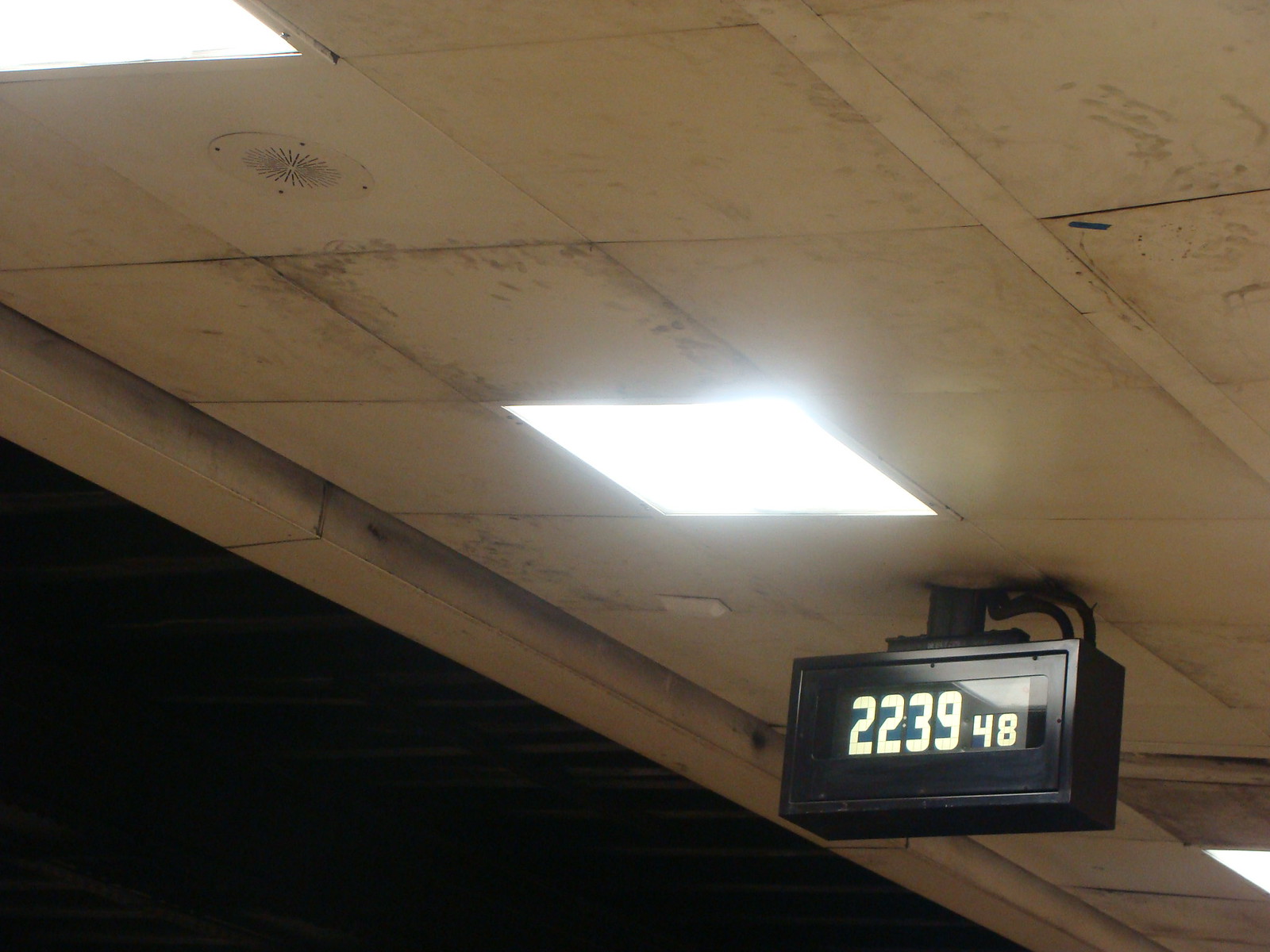The image appears to capture an outdoor train or rail station during nighttime. The primary focus is on the ceiling of the station, which is composed of white tiles that are heavily caked in dirt and grime. Fluorescent lights are installed every three tiles, illuminating the area intermittently. A black, square clock is prominently featured, extending from the ceiling and displaying the time as 22:39:48, indicating it is 10:39 PM and 48 seconds. The dark, night sky is visible to either side of the image, reinforcing the late-hour setting.